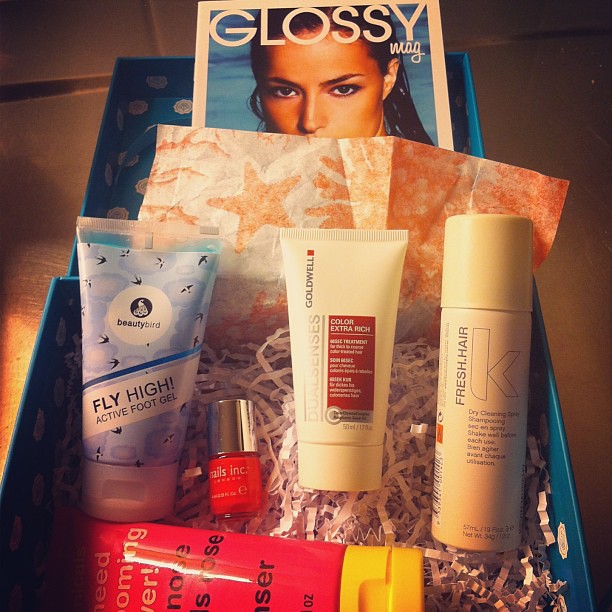An open blue box filled with shredded pink packing paper reveals an assortment of beauty products. Among the items, there is a red and yellow tube, a blue and white tube, and a "Beauty Bird Fly High Active Foot Gel" with a blue label and bird design. A small red-orange "Nails Inc." nail polish with a silver cap stands out alongside a "Dual Senses Extra Color Extra Rich" conditioner in a white bottle with a white top. Lastly, there’s a "Fresh Hair K" product in a white bottle. The box also includes an open magazine titled "Glossy Mag," featuring a woman by the beach staring directly at the viewer. The box is meticulously arranged to showcase the products, with decorative wrapping paper featuring coral and starfish patterns adding a beachy vibe.